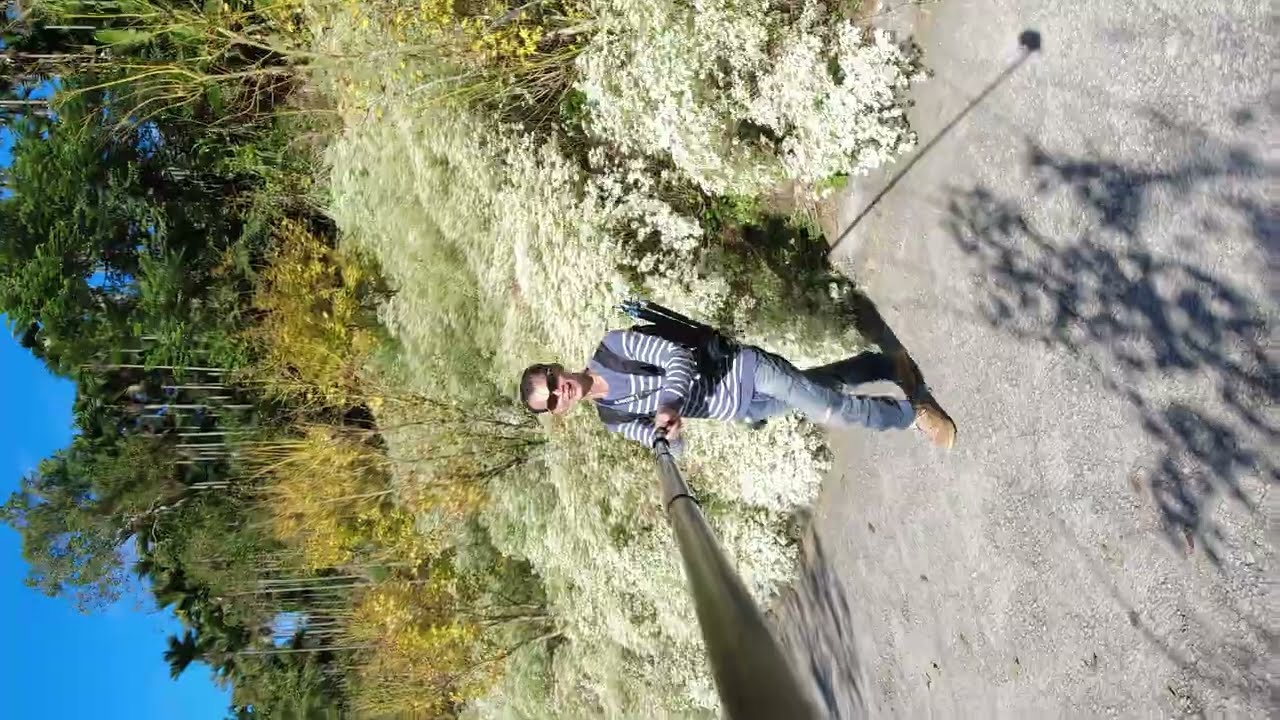A young Asian man, approximately in his early twenties, is depicted in this sunlit outdoor scene, captured from a sideways angle. He sports short brown hair and wears stylish sunglasses. His attire includes a blue and white striped sweater paired with blue Levi's jeans, notably featuring a hole at one knee, and sturdy walking shoes or boots. He is holding a selfie stick, positioning his phone or camera high above to take the selfie.

He stands on an asphalt pavement path that winds through a lush, sloped hillside. The background reveals a picturesque blend of natural elements: a clear blue sky, shadows cast on the path, and a variety of flora. Behind him, there are bunched white flowers with green shoots popping up among some weeds, small shrubs, and trees. Additionally, bamboo trees and other types of trees dot the hillside, cascading down towards the path he is walking on, hinting at a serene hiking trail in the wilderness. The bright sunlight and absence of clouds suggest the photograph was taken on a clear daytime, emphasizing the vibrant and peaceful ambiance of the setting.